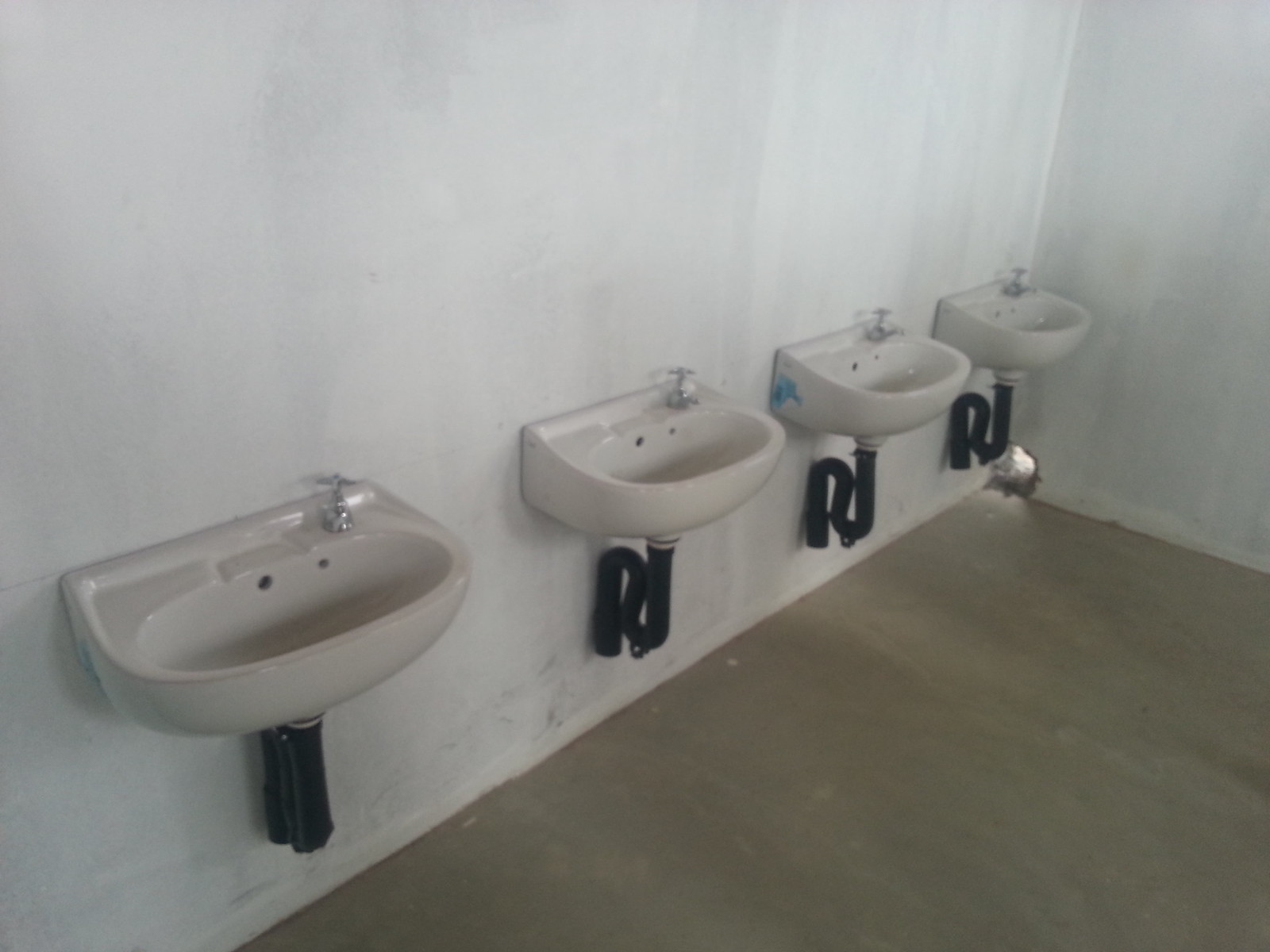This image captures the interior of a stark, minimalistic public restroom, possibly in a school, rest area, or even a prison. The bathroom features two white plaster walls and a barren, brownish-gray concrete floor. Four white porcelain sinks with single silver faucets on the right side are lined up against the main wall. The sinks are basic bowls with black S-shaped pipes coiled underneath, attaching them to the wall. Notably, one of the sinks has a small blue discoloration. There are no mirrors, soap dispensers, or paper towel holders—illustrating a severe lack of amenities and upkeep. In the corner of the room, near the floor, there's a hole where sunlight streams in, adding a touch of natural light to the otherwise plain and somewhat dilapidated space.